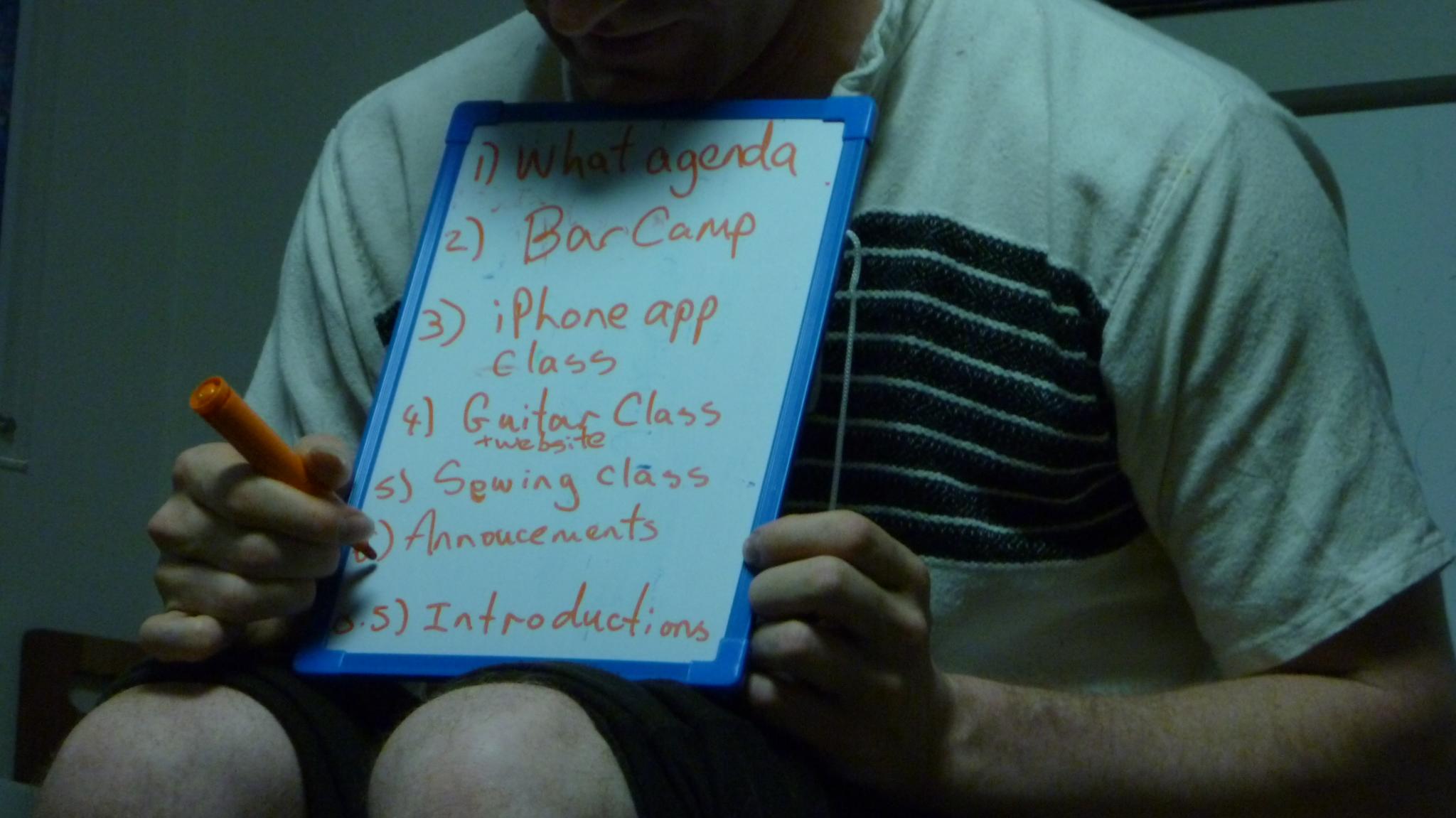In the photograph, a man, dressed in an off-white shirt with closely spaced dark stripes covering the middle of his chest, is seated. The image has a bluish-green tint, making the shirt's exact color somewhat ambiguous, but it appears tan or greenish off-white. His head is not visible in the frame. He is holding a whiteboard with a blue border between his chin and bare knees, as he is wearing shorts. In his right hand, he grips an orange marker, either writing or having already written on the board. The whiteboard lists several items in orange marker: "1. What agenda, 2. Bar camp, 3. iPhone app class, 4. Guitar class and website, 5. Sewing class, 6. Announcements," and at the very bottom, it reads "5.5. Introductions."